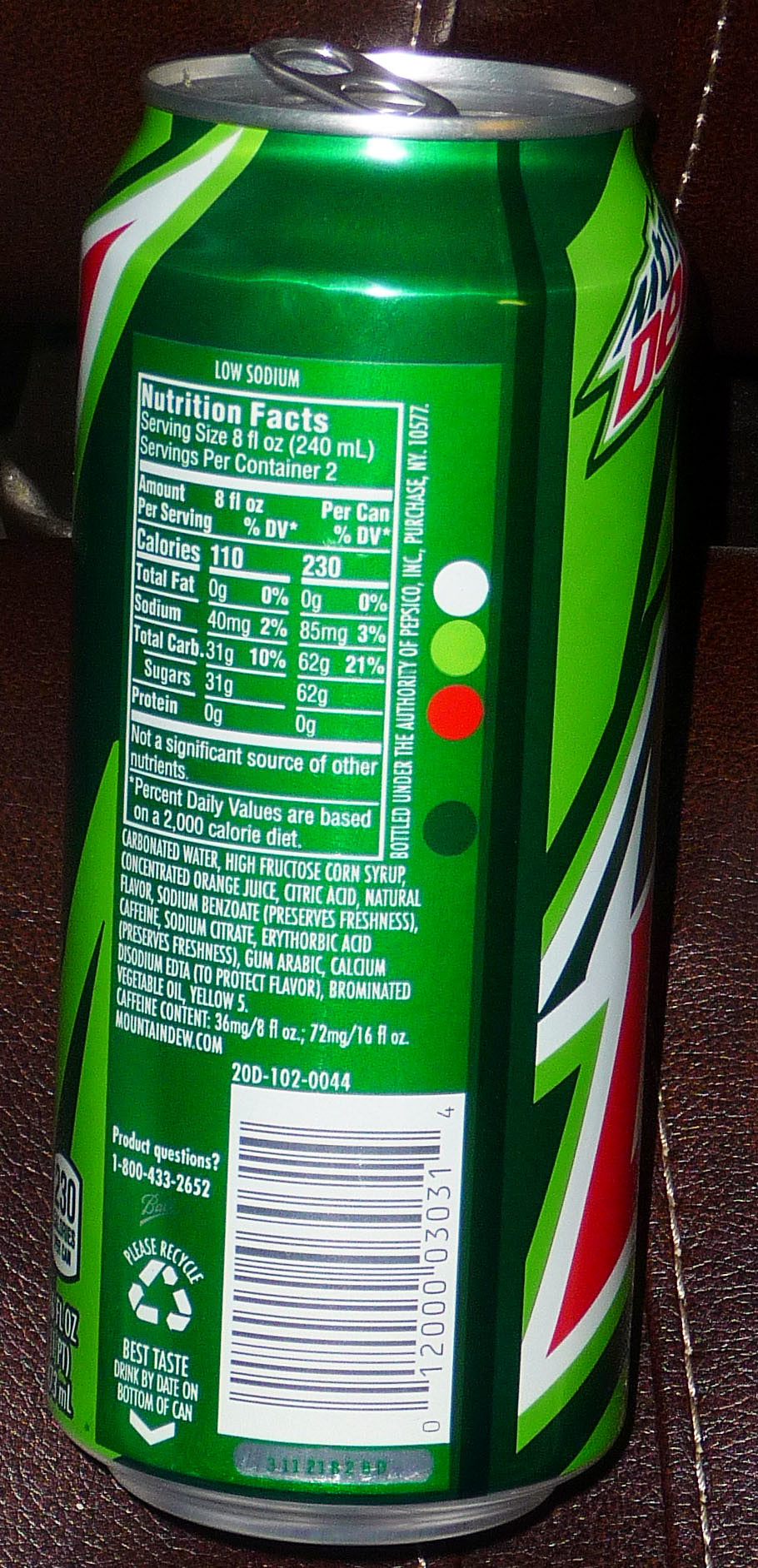A rich, dark-brown leather sofa, with subtle undertones of deep reddish hues, dominates the foreground of the image. Nestled on one of its plush cushions is a slim, small bottle of Mountain Dew. The bottle's label is clearly visible, showcasing detailed nutrition facts. Each serving size is noted as 8 fluid ounces (240 ml), with the bottle containing 2 servings. The nutritional breakdown per serving includes 110 calories, 0 grams of total fat, 40 mg of sodium, 31 grams of total carbohydrates, 31 grams of sugars, and 0 grams of protein. The photograph's composition draws attention to both the luxurious texture of the sofa and the crisp, informative label of the beverage.